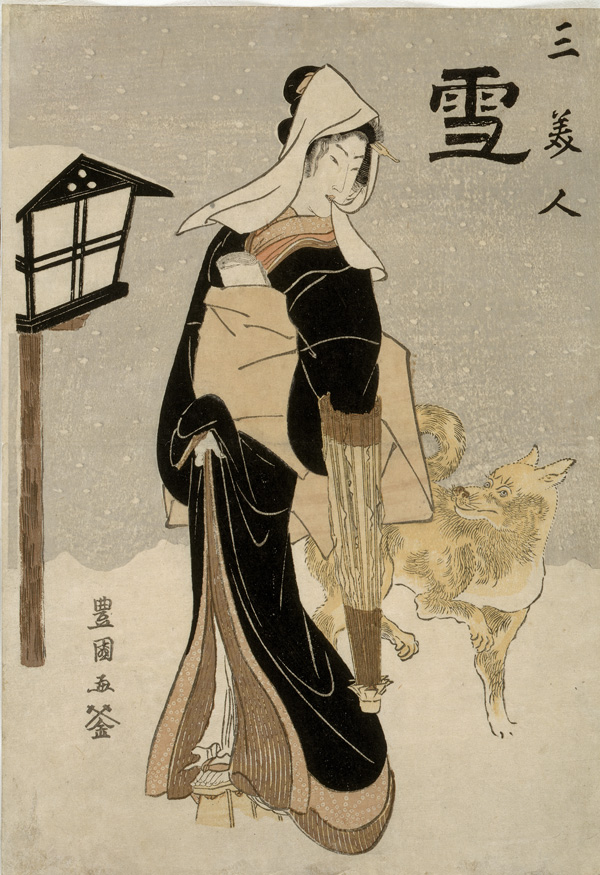A serene Japanese-style painting depicts a winter scene characterized by muted colors and intricate details. The backdrop features a snowy, gray sky dotted with white flakes, creating a calm and subdued atmosphere. In the upper right corner, elegant kanji characters are prominently displayed, possibly signifying a poetic or descriptive title. A further set of kanji runs vertically on the left side of the artwork.

In the foreground, a delicate and pale-skinned woman stands gracefully dressed in a flowing black and tan robe. Her black hair is neatly up, and she wears a white headscarf, a part of which she holds in her mouth. She dons traditional raised clogs, suggesting she is traversing a snowy path. Beside her stands a fox-like animal with orange fur and black markings, gazing intently at her, creating a sense of interaction. To her left, a distinctly Japanese light post or pole, adorned with a black-and-white structure reminiscent of a birdhouse, accentuates the traditional, tranquil setting.

Formulated with a blend of rich details from each observer, this composite description highlights the shared motifs and provides a vivid narration of the serene winter scene captured in this art piece.